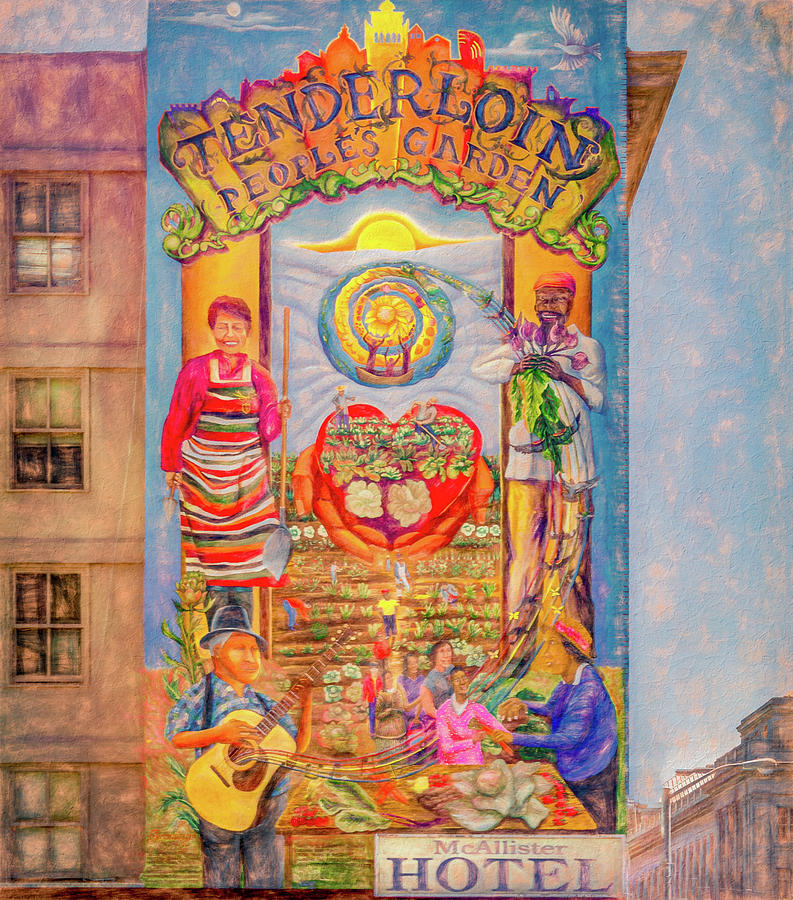The mural adorning the side of a three- or four-story building in a city or small town, prominently titled "Tenderloin People's Garden," bursts with vibrant colors and celebratory scenes. The top section features a sky-blue background with an orange band showcasing the mural's title in blue font. A torch, a symbol of hope and unity, is centered at the top with accompanying flowers, vines, and two orange pillars on each side. On the left pillar stands a middle-aged woman dressed in a multicolored, striped apron, holding a shovel in her left hand. On the right is an African-American man with red hair, holding a plant with leaves, possibly beets. Between them, a bright sun shines down with a circle of light radiating beneath it.

Below this, sets of hands cradle flowers and plants, symbolizing nurturing and growth. The garden scene below teems with activity. On the left is a man in a Peruvian hat, joyfully playing a guitar with musical notes streaming up towards the right where the man is holding beets. Centrally, people in indigenous costumes are vividly depicted gardening and harvesting vegetables, embodying a sense of community and connection to the land. On the right, a family is shown preparing food, capturing the essence of communal sharing. Completing the depiction, buildings with pink and gray windows frame the sides, with a dove appearing in the top right corner, symbolizing peace.

At the bottom-right corner of the mural, the name "McAllister Hotel" suggests that the building hosting this lively artwork may be the hotel itself. The overall scene exudes a happy, vibrant energy, emphasizing the unity and joy found in communal gardening and celebrating nature's bounty.